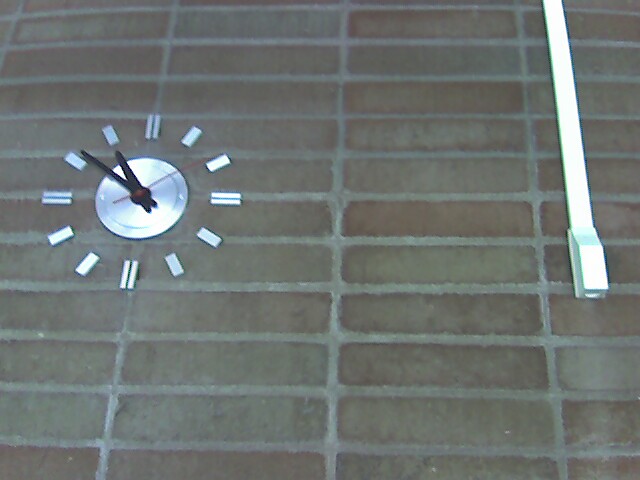This photograph captures an upward view of a large clock mounted on a brick wall. The brick wall features long, rectangular bricks in varying shades of red clay and tan, adding texture and visual interest to the composition. Positioned prominently in the center left of the image is a circular silver clock face. The clock face is bordered with evenly spaced double silver lines that represent the hours. A small red dot marks the center of the clock, from which black hour and minute hands extend, with a contrasting red second hand. On the right side of the photograph, descending from the top edge, is a thick silver line that terminates just past the halfway point of the image. The end of this line is notched, resembling a small grabber or hook, adding an additional layer of intrigue and complexity to the scene.